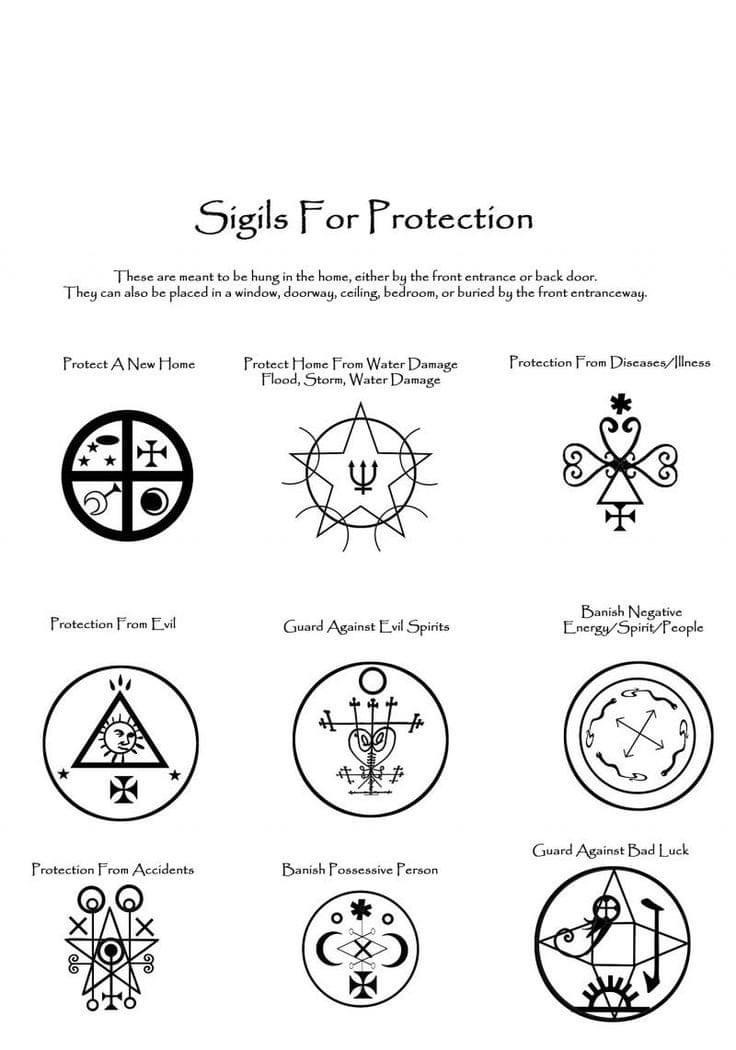The image is a detailed poster titled "Sigils for Protection," featuring nine distinct symbols arranged in a 3x3 grid. These sigils, designed to safeguard various aspects of a home, can be hung by the front entrance, back door, windows, doorways, ceilings, bedrooms, or even buried by the entranceway. 

Each symbol serves a unique protective purpose: 

1. **Top Left Symbol**: A circle divided by a cross into four sections, featuring stars and crescent moons, titled "Protect a New Home."
2. **Top Center Symbol**: A star encircled with additional half-circle pieces inside, inscribed "Protect from Water Damage, Flood, Storm."
3. **Top Right Symbol**: Swirly lines indicating "Protection from Illness."
4. **Middle Left Symbol**: Three circles with varying designs, one containing a triangle with a sun, labeled "Protection from Evil."
5. **Middle Center Symbol**: Hearts and lines signifying protection.
6. **Middle Right Symbol**: Additional symbol combinations for safeguarding different needs.
7. **Bottom Left Symbol**: Circles featuring crescent moons and diamonds.
8. **Bottom Center Symbol**: Varied shapes including stars and pitchfork-like elements.
9. **Bottom Right Symbol**: A symbol with a circle and intricate designs, marked with "Guard Against Bad Luck."

The poster showcases these symbols primarily in black ink against a white background to clearly delineate each detailed sigil. The text and symbols emphasize their intended protective functions, aiming to ward off various negative influences and ensure safety in the home.